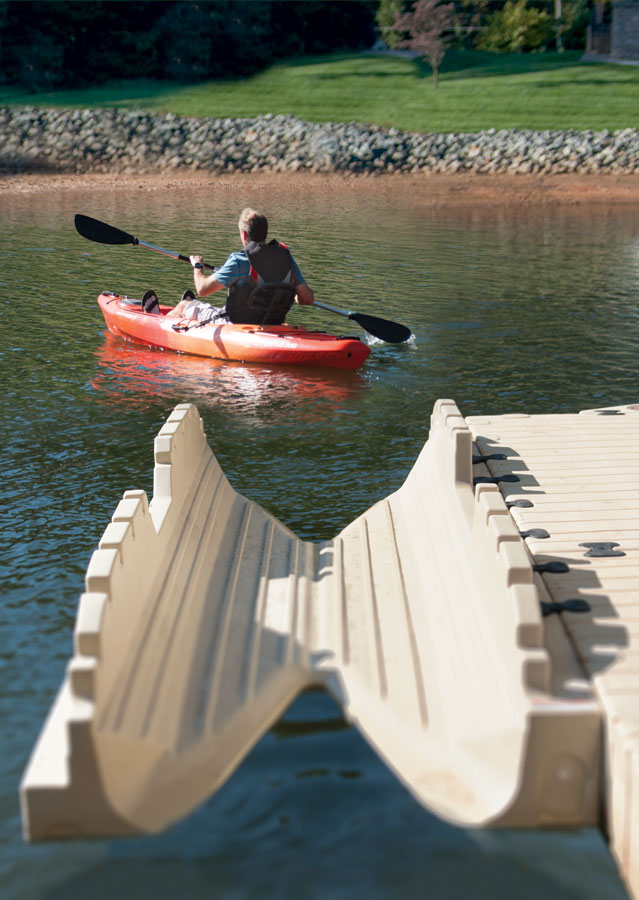A vertically aligned rectangular picture captures a serene lakeside scene featuring a man kayaking. The man is in an orange kayak, paddling diagonally to the left. He wears a blue short-sleeved shirt and appears to have short brown and gray hair. An oar, with its left side raised and the right side touching the water, spans the kayak. He may also have a life vest and a backpack. The water is a rippling grayish-brown.

The top of the image shows a partially blurry yet picturesque lawn with smaller trees and possibly a house in the distance. A low-level rock wall of uneven stones forms a boundary at the water's edge. In the bottom foreground, right in the center, is a beige-colored cradle or launcher designed to hold the kayak. It has grooves that fit the kayak's shape and is attached to a similarly colored dock, suggesting a practical setup for easy kayak storage. The dock and cradle appear to be made of plastic. The entire scene evokes the tranquility of a lakeside retreat, possibly a camp or reserve, with a lush green field adding to the natural beauty.